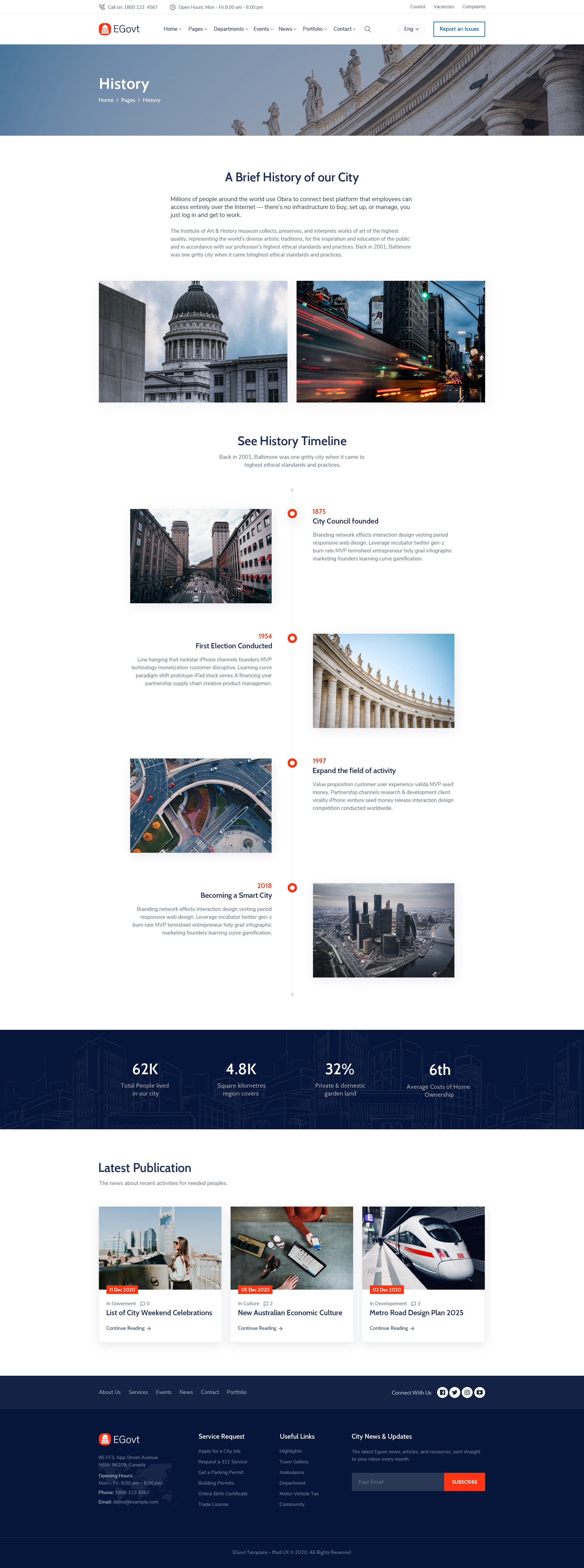Screenshot of a webpage titled "EGov" that appears to serve as a digital information portal for a city. The page prominently features a section labeled "History," which includes a brief historical overview and a video montage showcasing various landmarks of the city. Several images are displayed at the top of the page, including:

- An image of a historic Capitol building, suggesting the city's rich history.
- A structure with features reminiscent of a Coliseum, hinting at ancient architectural influences.
- A nighttime skyline shot of the city, illuminating its modern urban landscape.
- An aerial view of the city likely taken from a plane or drone, providing a comprehensive look at its layout.

The webpage also mentions a "see history timeline" link that presumably directs users to a detailed timeline of the city's history. Additionally, there are references to modern publications and a rapid transit system, indicating the city's blend of historical and contemporary elements. The page appears to offer an application for further city exploration, but the specific city's name remains unreadable due to small print.